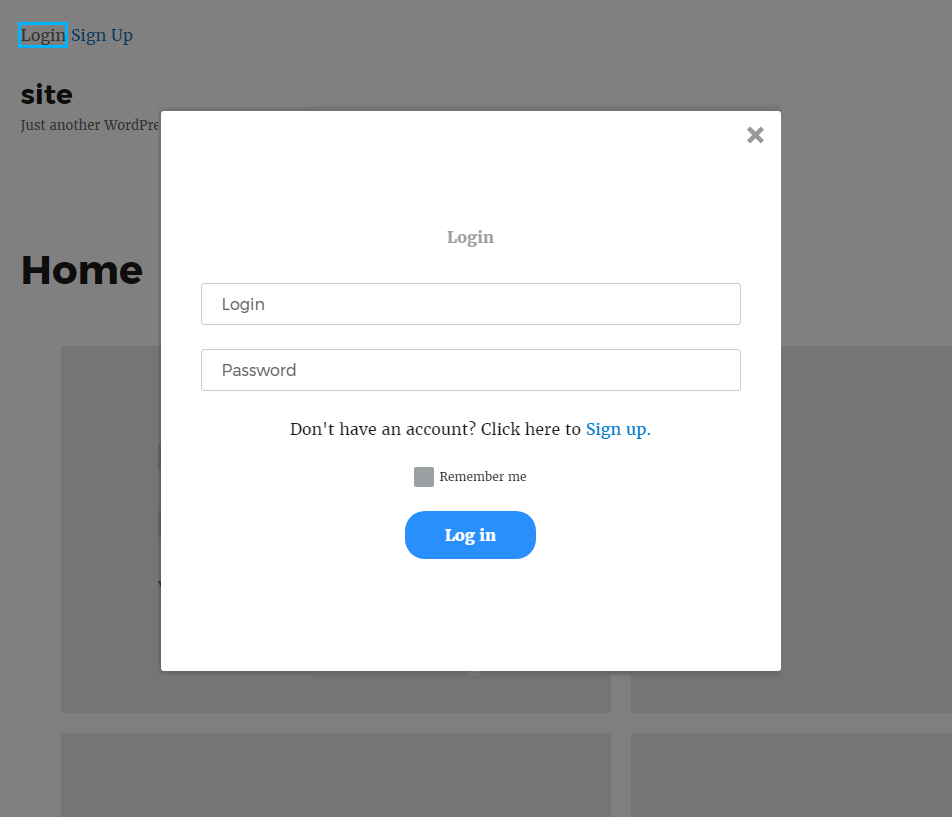A detailed and cleaned-up caption for the described image would be:

---

The image displays a sign-in page of an undisclosed website, presumably captured on a tablet or computer given the screen size, which is larger than that of a typical mobile device. The background is predominantly white, featuring basic design elements with minimal color. Central to the page are the options to either log in or sign up, alongside the phrase "Just another WordPress site" – suggesting that the page was created using WordPress, a well-known website creation platform. In larger font, the word "Home" is visible. The user seemingly clicked the "Login" button, which brings up fields for entering a username and password. There is also a "Remember Me" option for ease of future access. The overall design is very straightforward and lacks distinctive features or detailed information about the site's purpose, possibly due to content being blurred out or not yet loaded until user authentication.